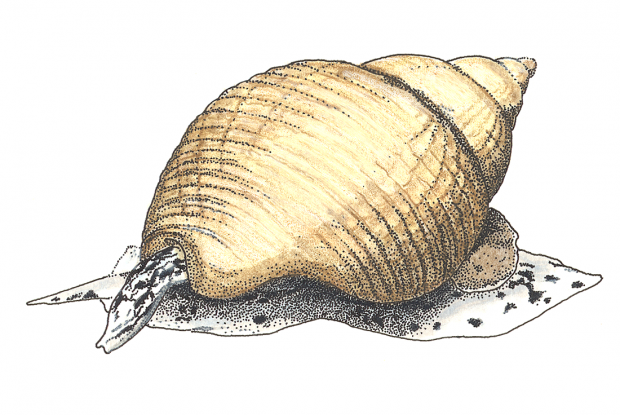This color illustration, likely hand-drawn, is of a snail emerging from an elongated, spiral shell, set against a stark white background. The shell is a pale golden yellow adorned with intricate patterns and texturing created by brown, dark brown, and black pencil lines, giving the impression of a corrugated surface. The shell, which appears to be facing the viewer, houses a predominantly white mollusk marked with black specks, suggesting either a land snail or a marine creature. Despite the simplicity of the drawing, which might evoke the style of a child's artwork, the image captivates with its blend of beauty and functionality, showcasing the shell as both an attractive object and a secure home for the living creature inside. The snail's head or antennae emerge from beneath the shell, directed to the left, adding a sense of life and motion to this otherwise static depiction.